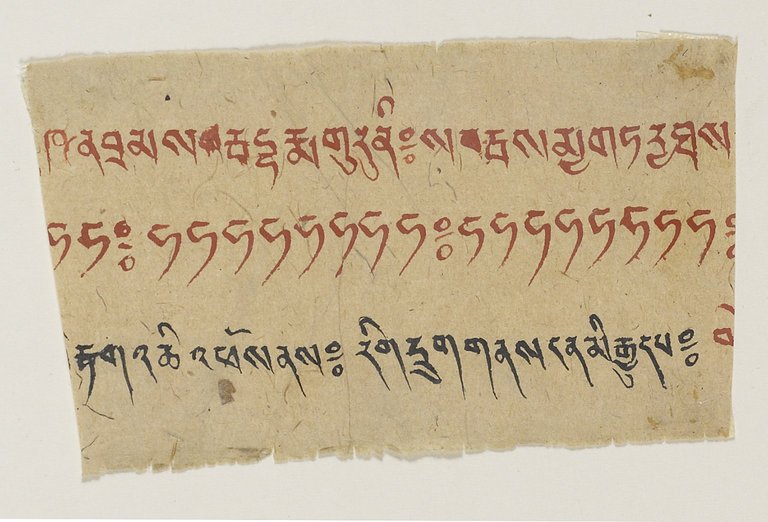The image features a beige, old piece of parchment paper, approximately six inches wide and four inches high, with ragged edges at the top and bottom suggesting wear and age. The left and right sides of the parchment appear slightly folded, giving them a crisper, more defined look. The background is a light gray with a muddy, brownish tinge that complements the old, weathered appearance of the parchment.

The parchment bears three rows of text, written in what appears to be Hindi or a similar script, though some descriptions suggest it could be Arabic or another language. The top two rows are written in red ink or paint. The first row contains symbols that look like a blend of letters and numbers, including shapes resembling the number two, five, and three, and what appears to be a percent sign. The second row predominantly features symbols that closely resemble the number five, interspersed with division symbols or percent signs. The third and bottom row is written in dark ink, either black or dark navy blue, but it features no recognizable pattern or description.

Additionally, the parchment has noticeable imperfections: a dark brown smudge near the bottom of the image and another smudge at the top right corner, adding to its aged and worn appearance.